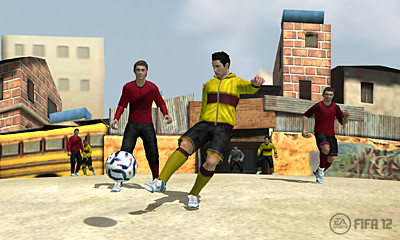In this vibrant scene from a computer game, the lower right-hand corner features a circular emblem that resembles the FIFA logo, and it possibly reads "82" or "12," though the text is somewhat obscured. Central to the image are two football players engaged in action. One player, clad in a red jersey and black shorts, competes against another dressed in a yellow jersey with a black stripe, black shorts, and yellow socks. Both are focused on a white soccer ball adorned with black patterns, ready to make their next move on what appears to be a paved playing surface.

The backdrop showcases a greyish-blue sky dotted with soft clouds. Prominent in the left background is a white building partially obscured by a red brick structure in the foreground. To the right stands a tall red brick building with a distinctive blue roof, accompanied by a smaller white building with a black roof. Amidst these structures are several yellow objects, potentially school buses or perhaps elements of a field. Just right of center, another player in a red football jersey and black shorts is visible, adding depth to the lively urban sports scene.